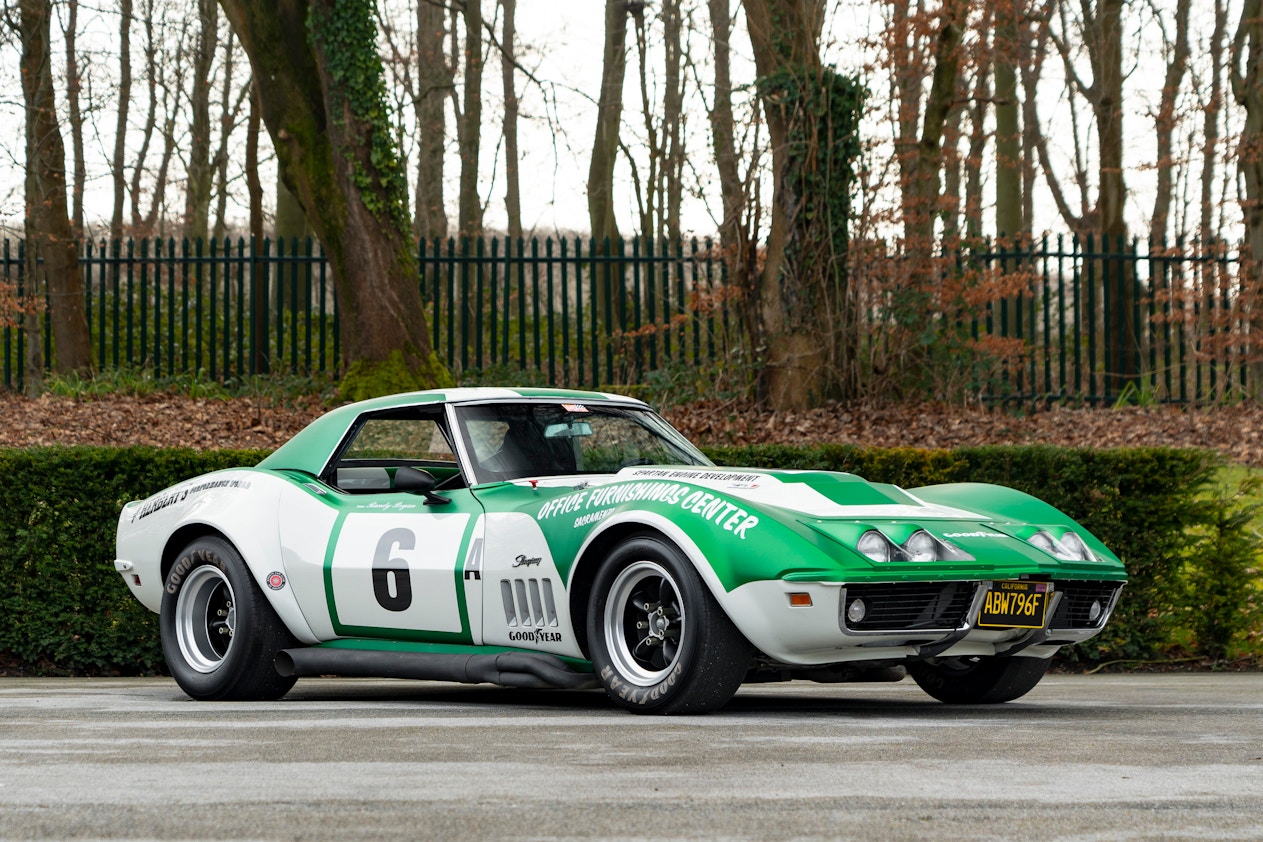This detailed landscape-oriented color photograph features a classic Chevrolet Corvette sports car prominently positioned in the center of the image, closer to the bottom. The vehicle is angled with its front end facing the bottom right corner and the rear positioned towards the lower middle section on the left. The car's bold, bright green body contrasts with its white rear quarter panel and black letterings. A significant detail is the large black number "6" displayed on a white rectangle on the side door.

The car's green roof and front fender are notable elements, the latter featuring the text "Office Furnishings Center" in all capital, white letters arcing over the tire well. Below this text is a Stingray decal with the Goodyear logo further down. The black tires have raised white letters with the Goodyear logo prominently visible. The vehicle’s striking green hood houses four round headlights at the front.

The car's license plate reads "ABW 796F" in yellow on a navy blue background, and it states "California." This is attached to the front right side of the vehicle. The backdrop showcases a green hedge beneath a black fence and several dead trees with a bright, white sky overhead. The car is parked on gray pavement, creating a stately yet realistic representation of this vibrant sports car.